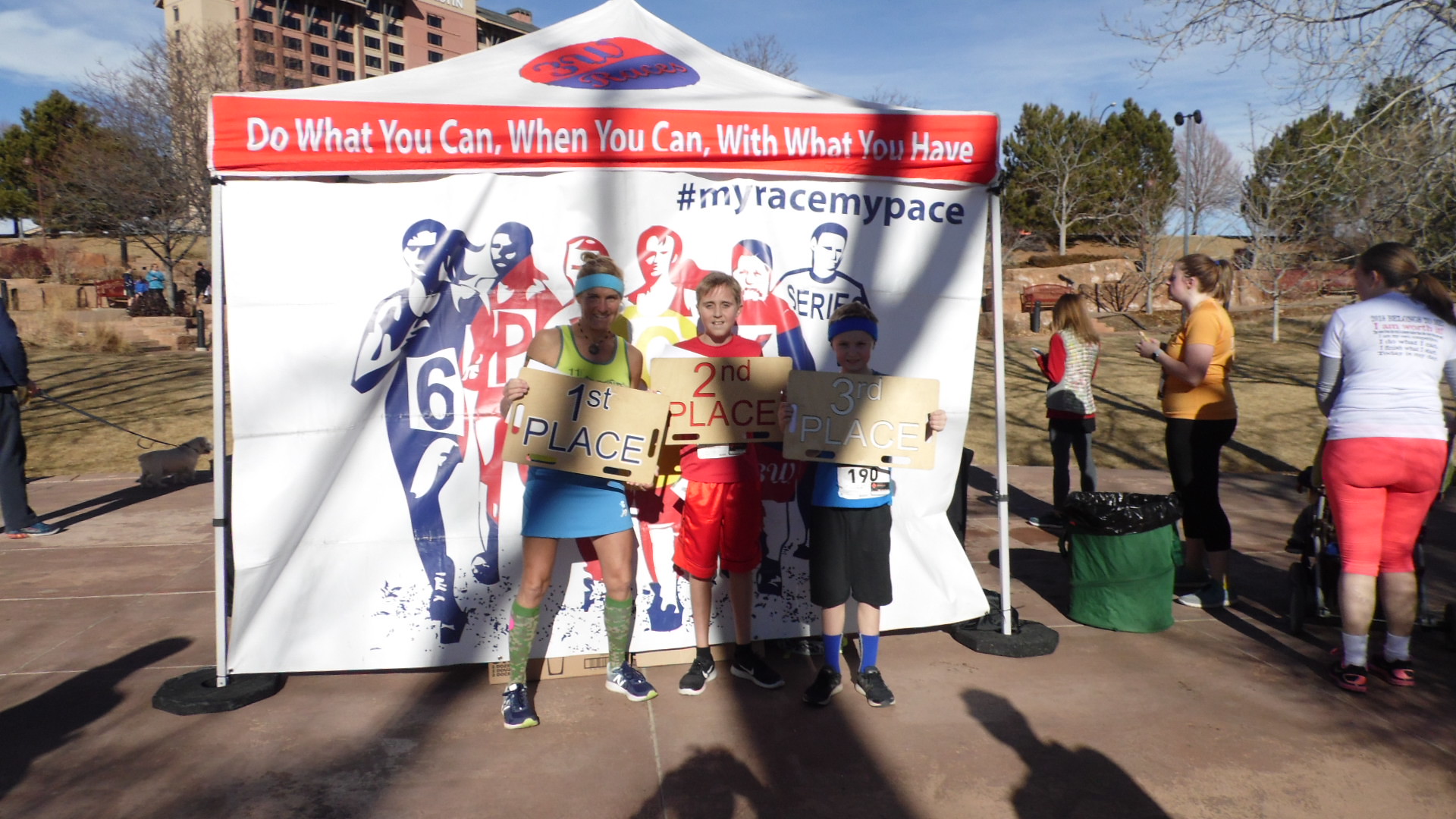In an outdoor park-like setting, this rectangular photograph captures a lively race event. Central to the image are three individuals standing in front of a large banner attached to an outdoor tent. The banner prominently displays the motivational message, "Do what you can, when you can, with what you have. #MyRaceMyPace," along with shadowed figures in the background. 

The three individuals, posing for the photograph, hold signs indicating their placements: first place, second place, and third place. The first-place participant, an older woman wearing gym shoes and athletic attire, stands beside two younger boys who secured the second and third spots. Behind them, a high-rise building, likely condominiums or apartments, reaches toward the sky, emphasizing the urban backdrop.

The race participants are dressed in running gear such as leggings and shorts, with some wearing brightly colored shirts—red, orange, and white. A few additional details in this dynamic scene include a green garbage bin nearby and a mix of trees, pavement, and background objects like a garbage van and people with their backs turned, further enriching the photograph's narrative.